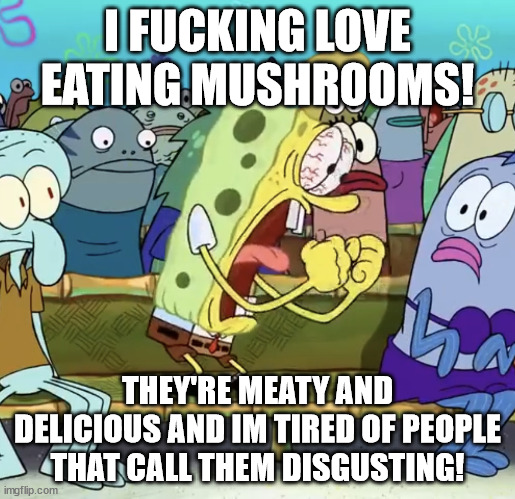A meme image using a scene from the cartoon "SpongeBob SquarePants" features SpongeBob in a state of intense emotion. Text at the top exclaims, "I fucking love eating mushrooms!" SpongeBob is depicted in the middle of a vigorous outburst, eyes bulging and fists clenched as he screams, surrounded by other characters who look on in shock, their eyes wide with surprise. The text at the bottom reads, "They're meaty and delicious, and I'm tired of people that call them disgusting." This meme humorously addresses the divide in opinions about mushrooms, highlighting the author's passionate preference for their unique texture and flavor.